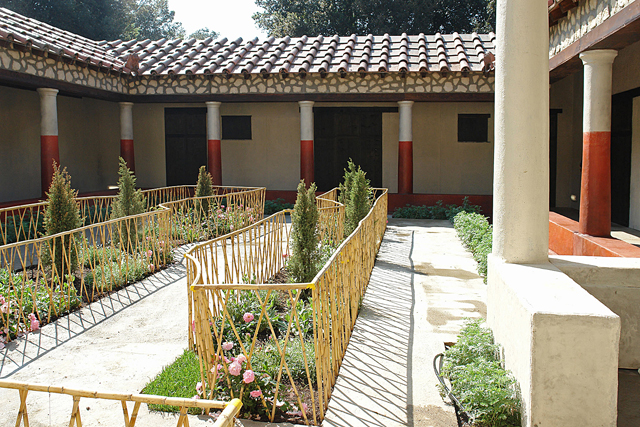This photo captures a unique, enclosed outdoor area that appears to be part of a house or perhaps a hotel, given its numerous entrances and rooms. The structure is reminiscent of a small, one-story home that wraps around a central courtyard, forming a square or rectangular shape. The building itself is beige with distinctive posts painted in red and white, and the roof appears to be made of clay or concrete. The courtyard, accessible via gray cement walkways, features a lush garden with a variety of plant life, including pink flowers, arborvitaes, and small bushes. Additionally, white and goldish fences enclose some of the garden areas, creating sections with miniature trees and grassy patches. Sunlight illuminates the scene, further enhancing the vibrant colors of the garden's flora.